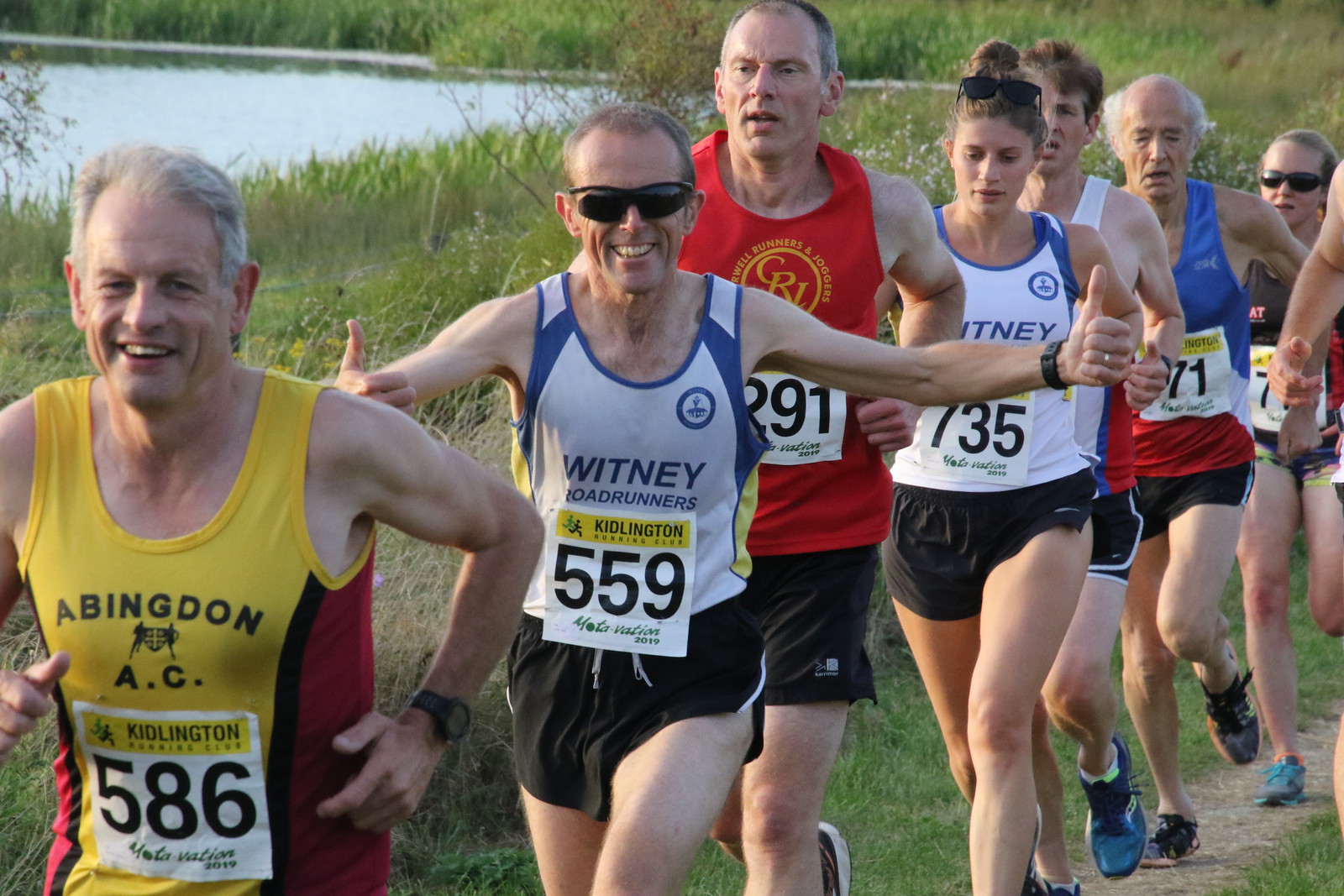In an outdoor setting during the daytime, a group of runners is captured mid-race on a dirt trail winding through a grassy area with a lake and tall vegetation in the background. Leading the pack is a smiling gentleman in his 50s or 60s, with graying hair, wearing a yellow and blue jersey with the number 586. Behind him, a man in a white and blue sleeveless tank top with black shorts, marked with bib number 569, stretches his arms out in a thumbs-up gesture, sporting black sunglasses and a watch on his left wrist. Trailing them is a man dressed in a red jersey and black shorts, labeled with the bib number 291. Following closely is a woman in a white and blue jersey with black shorts and sunglasses perched atop her head, wearing bib number 735. Further back, another runner in a white and red shirt and black shorts has a partially visible bib. Among the runners, there is also a man in a red, white, and blue shirt with the bib number 71 and a woman in a black shirt with glasses, whose bib is obscured. The diverse group, seemingly at various levels of exhaustion, runs in a roughly single file along the well-trodden path.